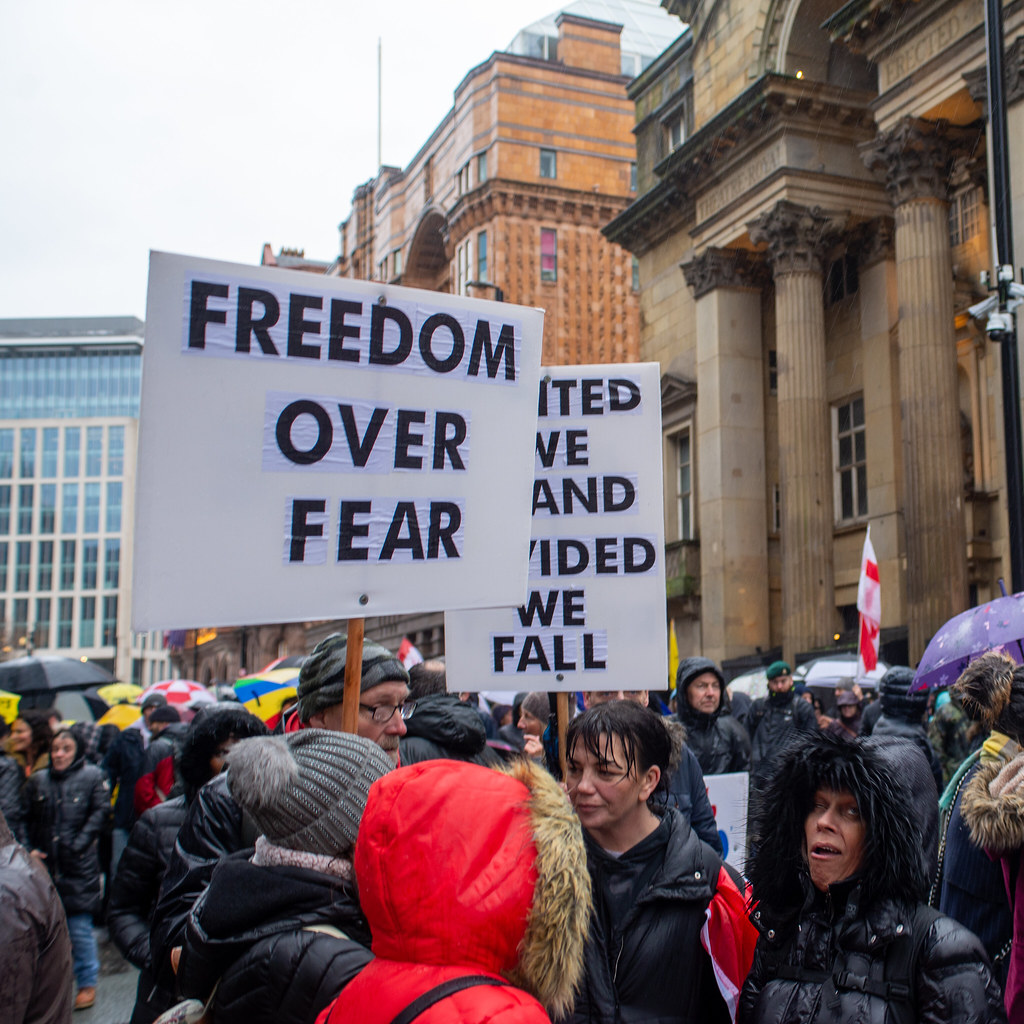In this photograph, we see a daytime outdoor protest or demonstration in a city, taking place in front of old stone buildings with prominent stone columns. The weather is cold and rainy, as evidenced by people dressed warmly in coats and hoods, with wet hair and numerous umbrellas of various colors, including black, red, and a multicolored one with green, blue, yellow, and red panels. The sky is mostly cloudy. The participants appear to be of Caucasian descent. 

Two white rectangular signs with black lettering are prominently featured. The first sign, more portrait-oriented and closer to the viewer, reads "Freedom Over Fear." The second sign, partially obscured, likely says "United We Stand, Divided We Fall." A red and white flag is also visible among the crowd. In the lower right corner, a woman in a black fur-lined hood stands out, making a humorous face with her eyes rolled back and mouth open, providing a stark contrast to the serious atmosphere of the protest. The overall color palette includes shades of white, tan, black, and red.